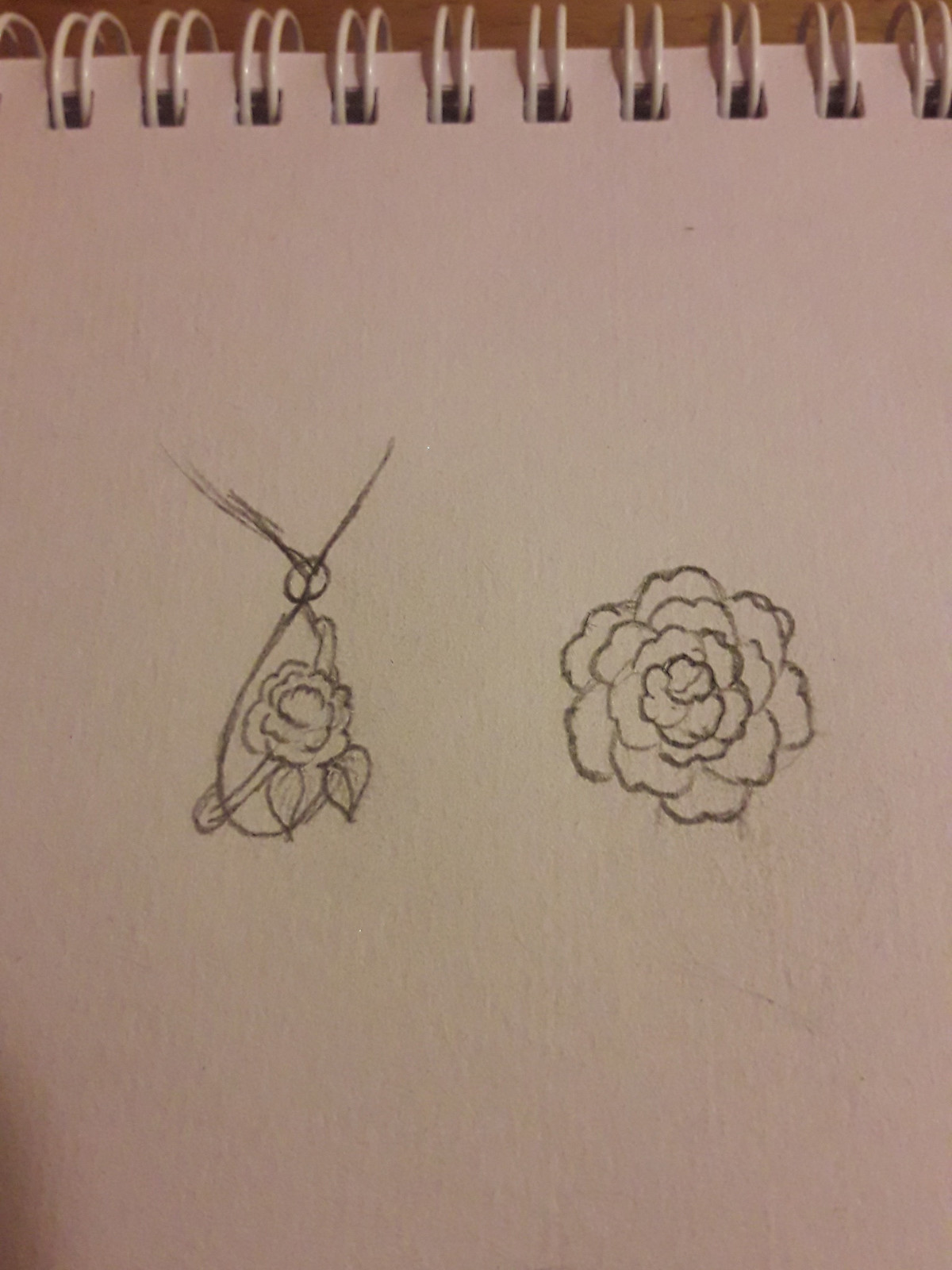A detailed view of an artist's spiral sketchbook is captured in this image, showcasing intricate pencil sketches. The white spirals at the top run through small perforations, creating a clean, organized appearance. Toward the top left, a delicate sketch portrays a rose pendant hanging from a necklace. The pendant, teardrop-shaped with a detailed rose etched inside and encircled by a ring, is attached to V-shaped, shaded lines representing the necklace chain. Adjacent to this, on the right, is a meticulous pencil drawing of a rose with numerous layered petals, emphasizing the artist's skill in capturing delicate details.